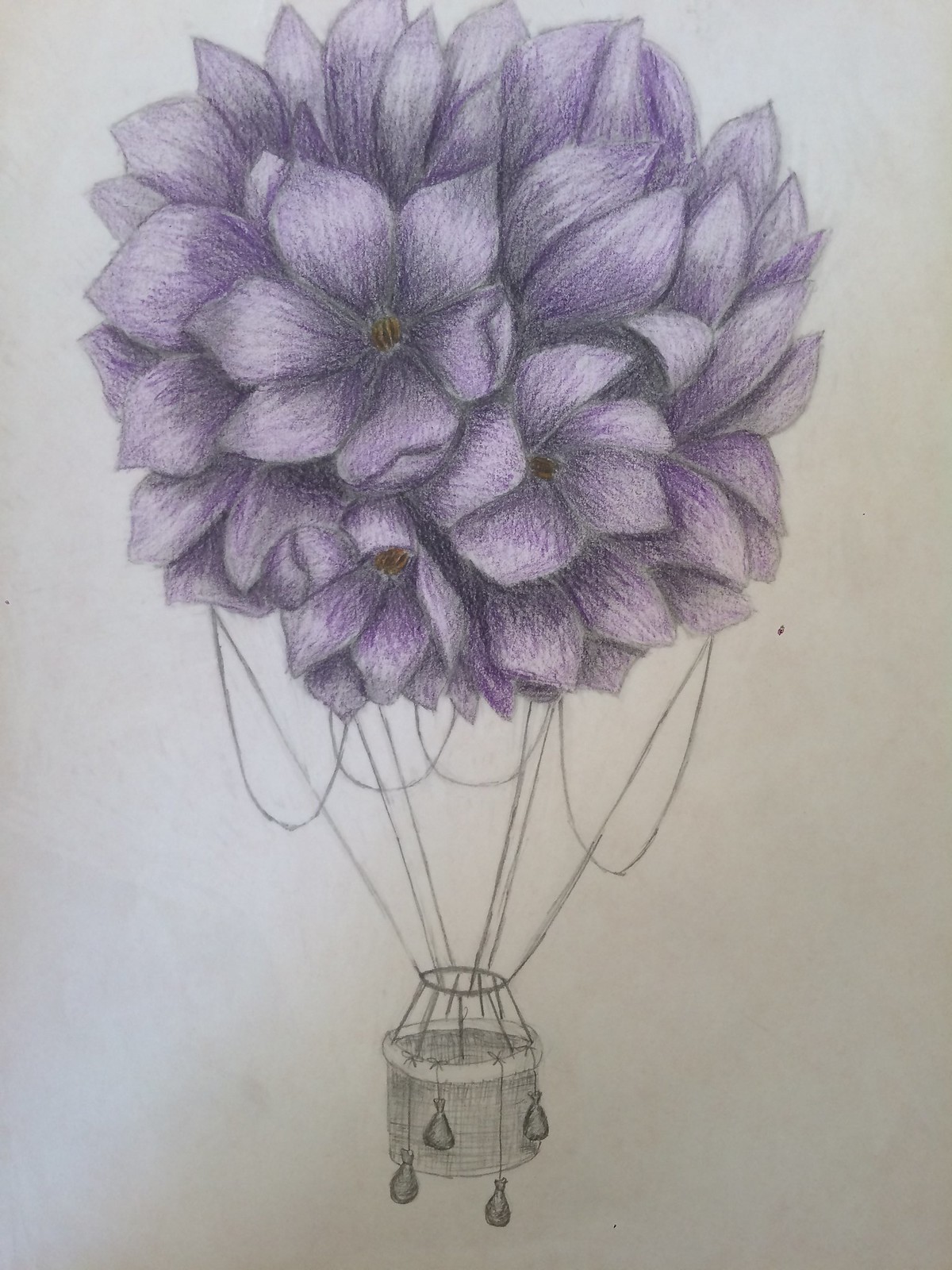This is a detailed hand-drawn image on slightly yellowed white paper, depicting a fantastical hot air balloon. Instead of the typical balloon, the top is formed by a bouquet of purple flowers, which resemble daisies. Each flower has six purple petals with white shading, and their centers display a striped yellow and black pattern akin to bee markings. The flowers are in various stages of bloom, some fully open and others still budding, collectively creating the spherical shape of a traditional hot air balloon.

The balloon is tethered to a woven basket below, reminiscent of an Easter basket, which acts as the carriage. The basket is detailed with a railing and four small sandbags hanging from its sides for ballast. Connecting the basket to the balloon is an intricate network of strings and metal supports, looping and crisscrossing downwards from a central ring towards the basket. The background of the image is a dull gray, offering a muted contrast that highlights the vibrant bouquet at the top. This whimsical illustration combines elements of nature and classic hot air balloon design into a unified and imaginative scene.